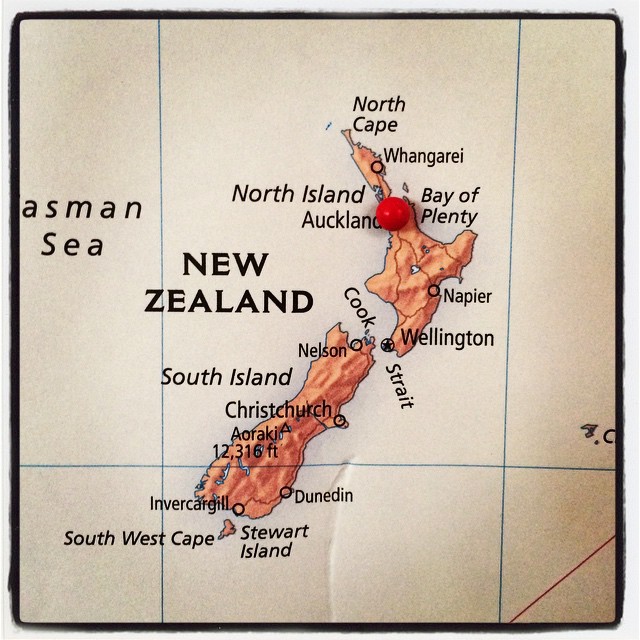This image is a highly detailed map of New Zealand, featuring a light brown background that resembles the color of paper, providing a distinctive and unusual visual style for a map. The map's focus is on New Zealand, prominently outlined in a reddish-orangish hue, and the surrounding Tasman Sea between New Zealand and Australia. "New Zealand" is inscribed in large black letters centrally on the map.

A red pin marks the location of Auckland on the North Island, which stands out with its label among other cities and landmarks noted across both North and South Islands. Noteworthy places included are North Cape, Whangarei, Bay of Plenty, Napier, Wellington, Nelson, Christchurch, Mount Aoraki, Dunedin, Invercargill, and Stewart Island with the Southwest Cape. The cities and points of interest are labeled in black text. This map not only highlights the central landmass of New Zealand but also provides a clear depiction of the surrounding seas and significant geographical points, making it an informative and visually engaging representation of the region.